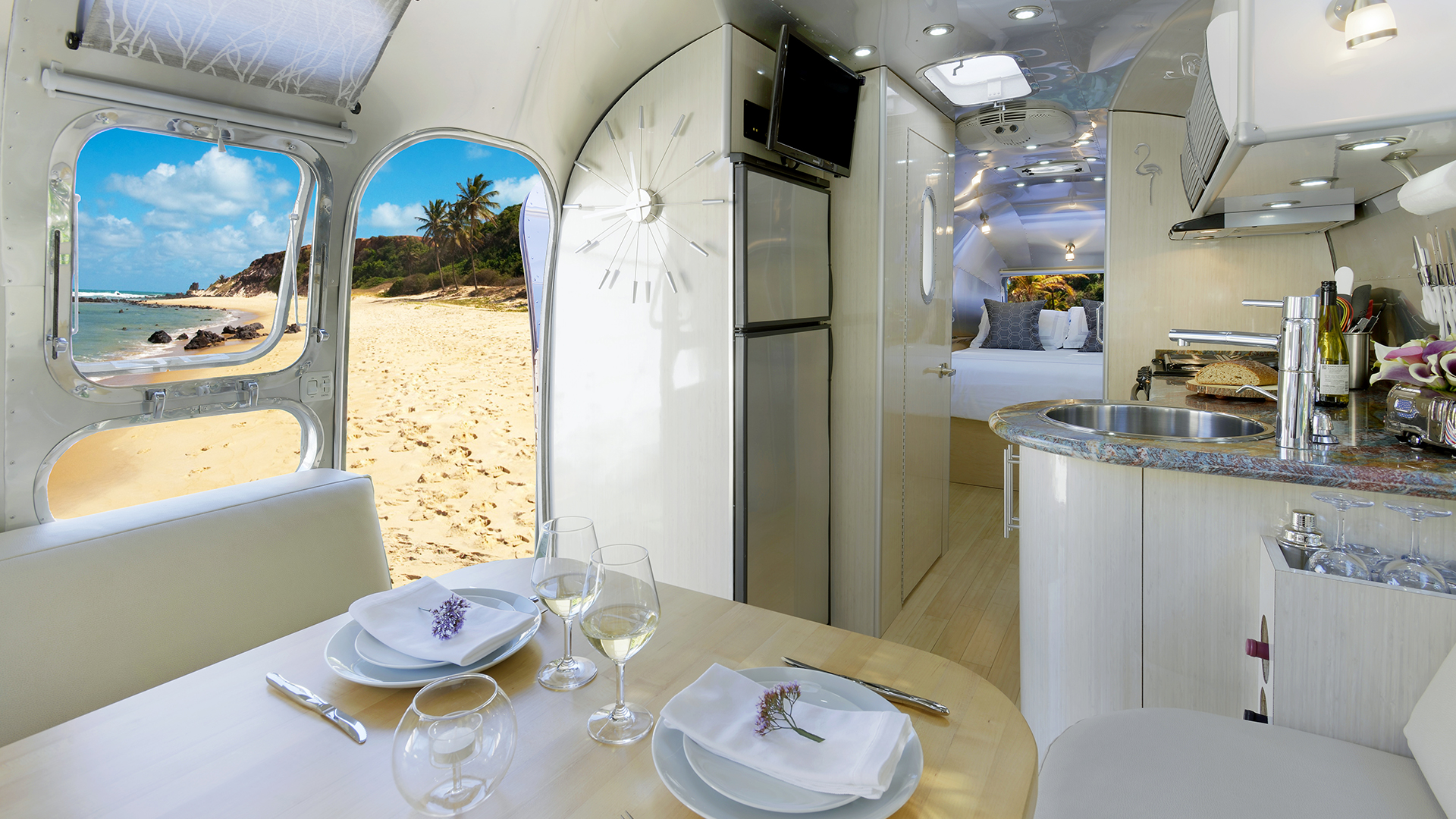The image showcases the sophisticated interior of a modern motorhome parked on a sandy beach. The walls and cabinets are pristine white, creating a sleek, futuristic ambiance. The cozy kitchen area on the right features a granite countertop with a loaf of bread, a silver fridge topped with a small TV, and an accompanying large clock. The bed, located centrally at the back, is adorned with white and gray pillows and a white blanket, resting beneath a skylight that adds natural light.

In the foreground to the left, a stylish dining area is set up with white seating, plates, silverware, and wine glasses filled with white wine. Each plate is garnished with a napkin and a small purple flower, adding a touch of elegance. The floor contrasts subtly in wood and beige hues.

Through the open door and window at the top left, the stunning outdoor scenery is visible, featuring a sandy beach, swaying palm trees and grass to the right, with the vast ocean stretching out to the left under a blue sky dotted with white clouds. This scene underscores the luxurious and serene setting of the motorhome.